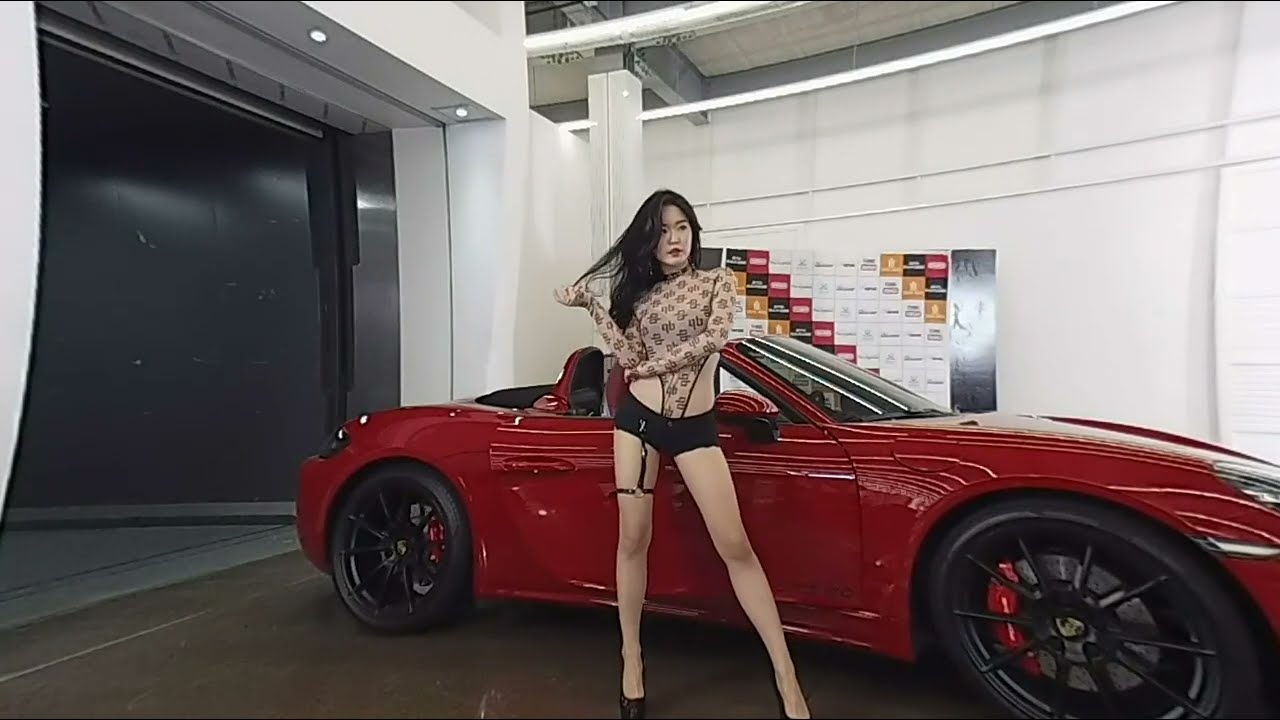In a well-lit showroom with a white backdrop and a brown stone floor, a striking East Asian model with long hair poses in front of a luxurious candy apple red Mazda Miata sports car. The car features black rims with ten spokes and a red frame around the slanted windshield. The model is dressed in a revealing light tan top adorned with dark brown designs, paired with extremely short black shorts and a leather garter adorned with metal circles above her knee. She completes her eye-catching look with high heels. The showroom setting includes fluorescent lighting on the ceiling and walls adorned with some kind of chart displaying white, red, black, and brown rectangles with indeterminate lettering, adding a commercial feel to the scene. A large garage door or elevator appears to the left, from which the car seems to have emerged. The model's right hand holds part of her hair while her left hand rests near her right arm, adding to the allure of the photograph.